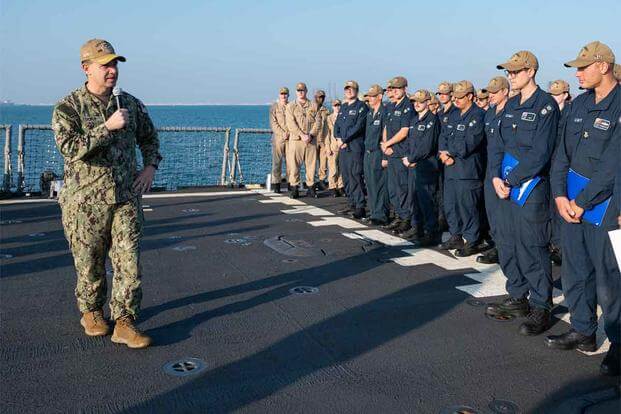In this image, taken on the deck of a Navy aircraft carrier under a clear, blue sky with no clouds, and the blue expanse of the ocean visible in the background, a group of personnel is assembled, standing behind a white line. Most individuals are dressed in blue Navy work clothes with black boots and khaki-colored baseball caps. Among them, some in the back are in khaki uniforms, also with tan hats. Centered prominently is a man clad in full camouflage fatigues, including a matching tan baseball cap and tan boots. He holds a microphone in his right hand, appearing to address and instruct the group, some of whom are holding notebooks, indicating a possible training session. The ship's railing is visible to the side, reinforcing the maritime setting.